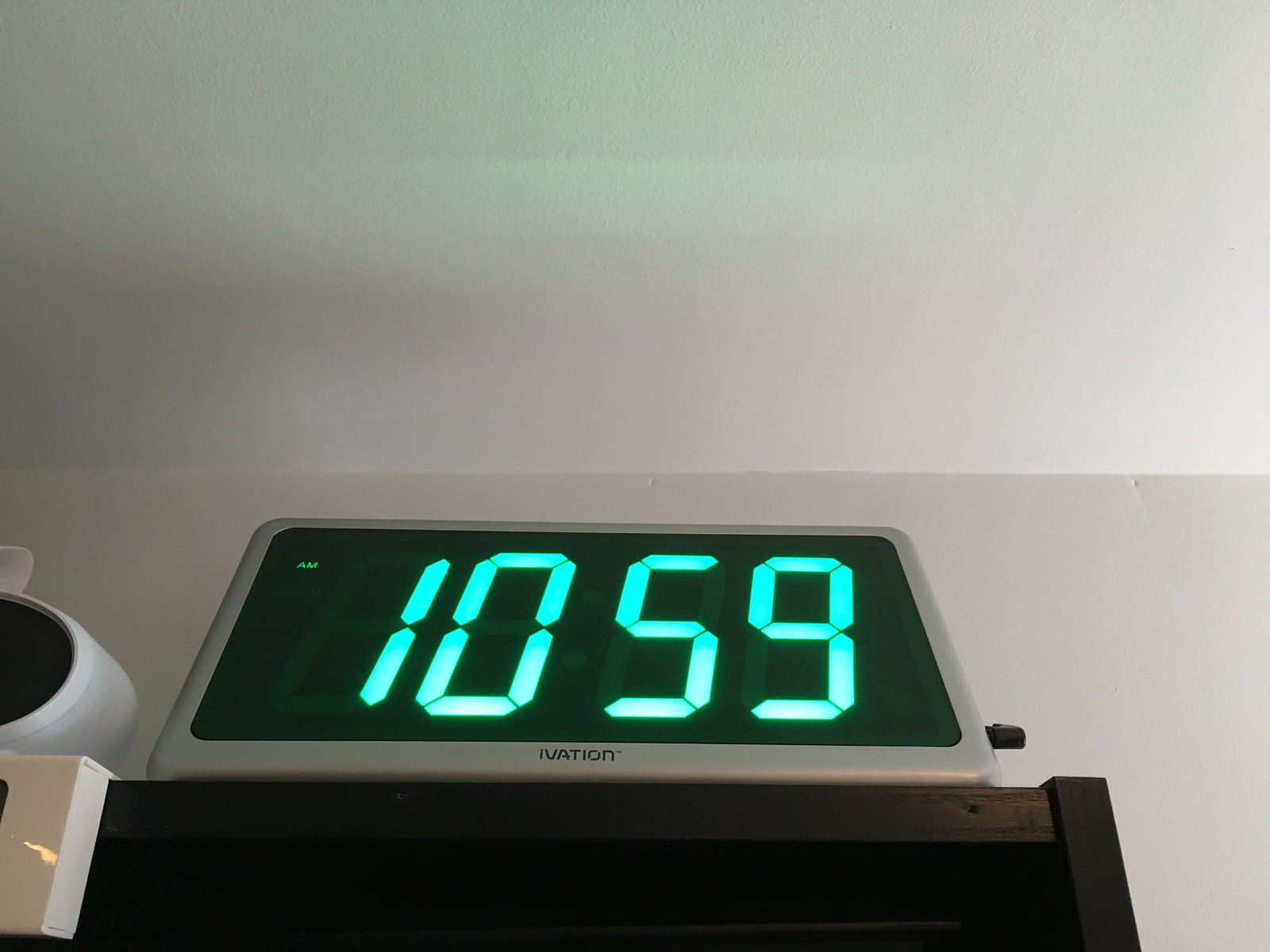The image depicts a modern alarm clock viewed from an upward angle, possibly suggesting that it is positioned on a tall shelf or that the perspective is from the floor. The ceiling and the adjoining wall, both immaculately clean and white, form the backdrop of the scene. The time displayed on the alarm clock is 10:59 AM, with large, easy-to-read digits illuminated in a greenish-blue hue. The clock’s outer casing is a sleek silver color, branded at the bottom with "IVATION." On the right side, a black nodule, likely a connection port or power plug, extends from the clock. The clock rests on a dark wooden stand. To the left of the clock, there is a small, white, circular plastic item, and attached to the front of the wooden shelf beneath them is a rectangular white plastic object.